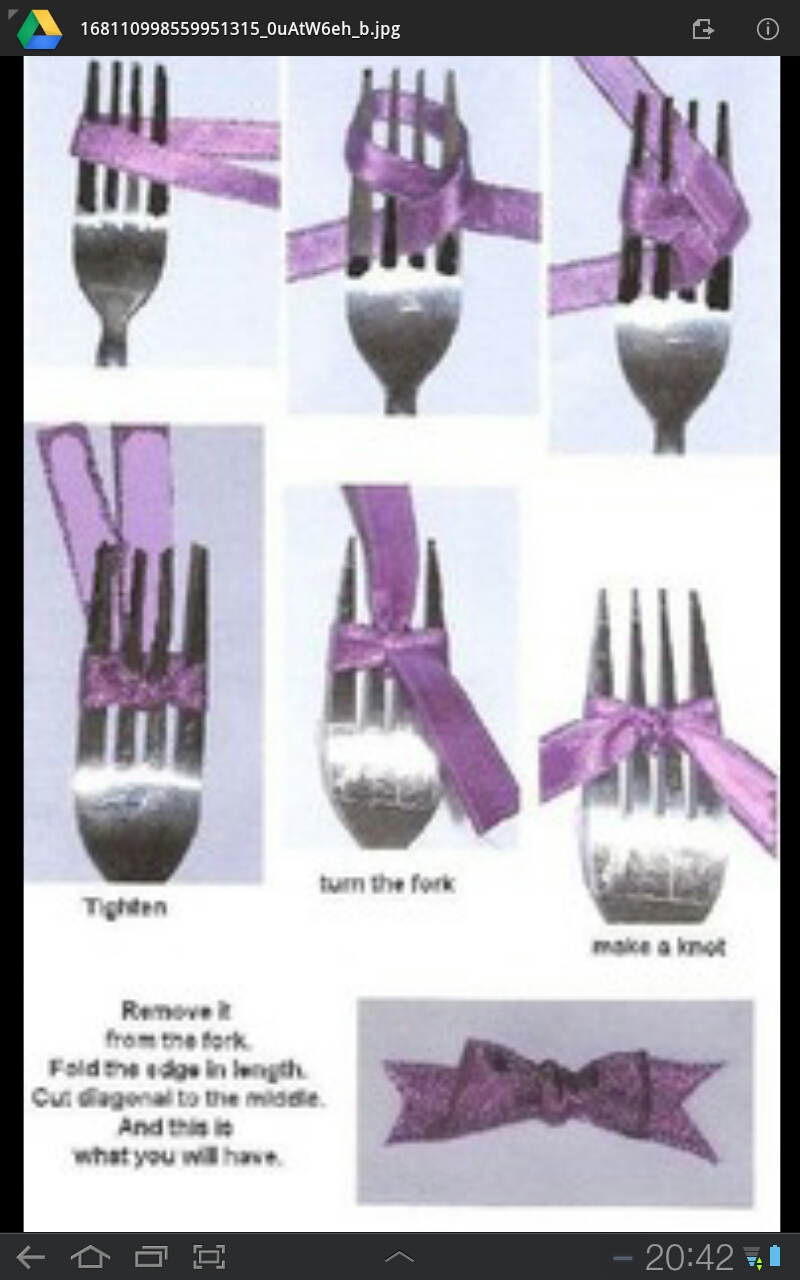This image, which appears to be a low-quality screenshot taken from a phone, showcases a step-by-step tutorial on creating a knotted bow using a fork. The screenshot has a black border and visible phone interface elements, including a Windows symbol in the upper left corner, a lengthy file name ending in ".jpg," and various icons such as a download option and a help exclamation point.

The primary content of the image consists of six sequential photos of a silver fork being used to create a decorative bow. The fork displays a series of steps for tying a bow with a ribbon, which is depicted in purple. The instructions detailed in the images read: "tighten, turn the fork, make a knot, remove it from the fork, fold the edge and length, cut diagonal to the middle," ultimately resulting in a delicate purple bow.

The images meticulously demonstrate the progression of steps needed, ensuring viewers can replicate the bow using the illustrated technique.